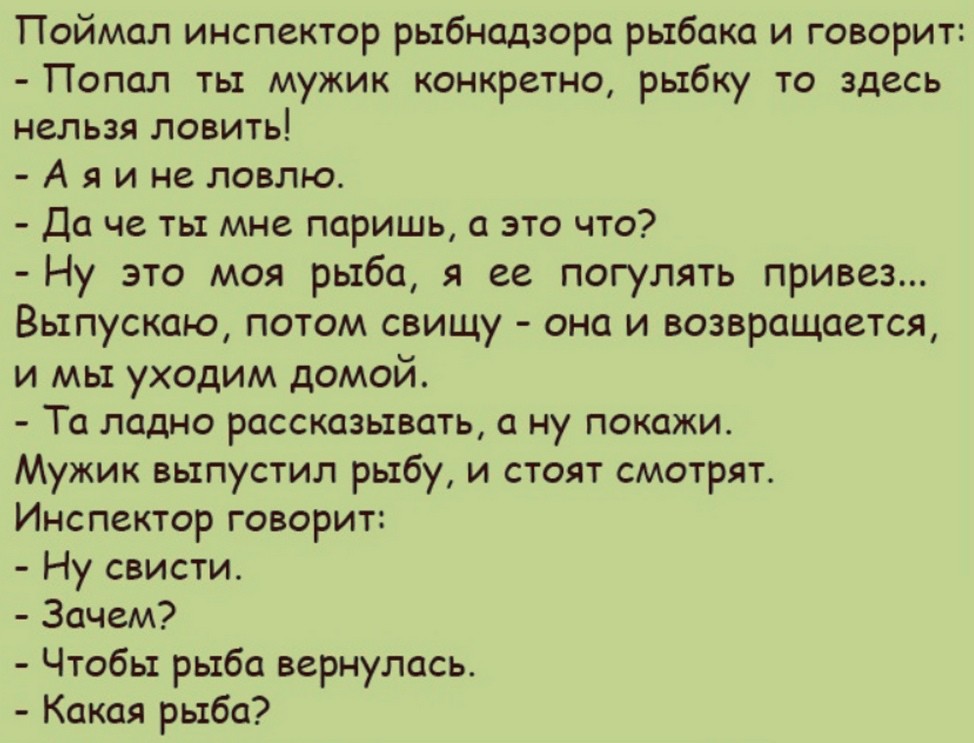The image is a wide rectangular block of text set against a pale green or pastel green background, resembling a board, poster, or display. The text is written in a dark color, either black or very dark brown, and appears to be in a non-English language, possibly Greek or another foreign script. The layout starts with several very long words at the top, ending with a colon. Following this is a series of lines: the first of which ends in an exclamation mark after spanning two lines of smaller words; next is a short sentence, then a slightly longer question, and a very long sentence that stretches across three lines and includes an ellipsis in the middle. This is followed by another very long sentence and another one that ends in a colon with a list beneath it. The pattern continues with multiple lines, alternating between full stops and question marks, with the text arranged neatly across approximately 12 to 13 lines.